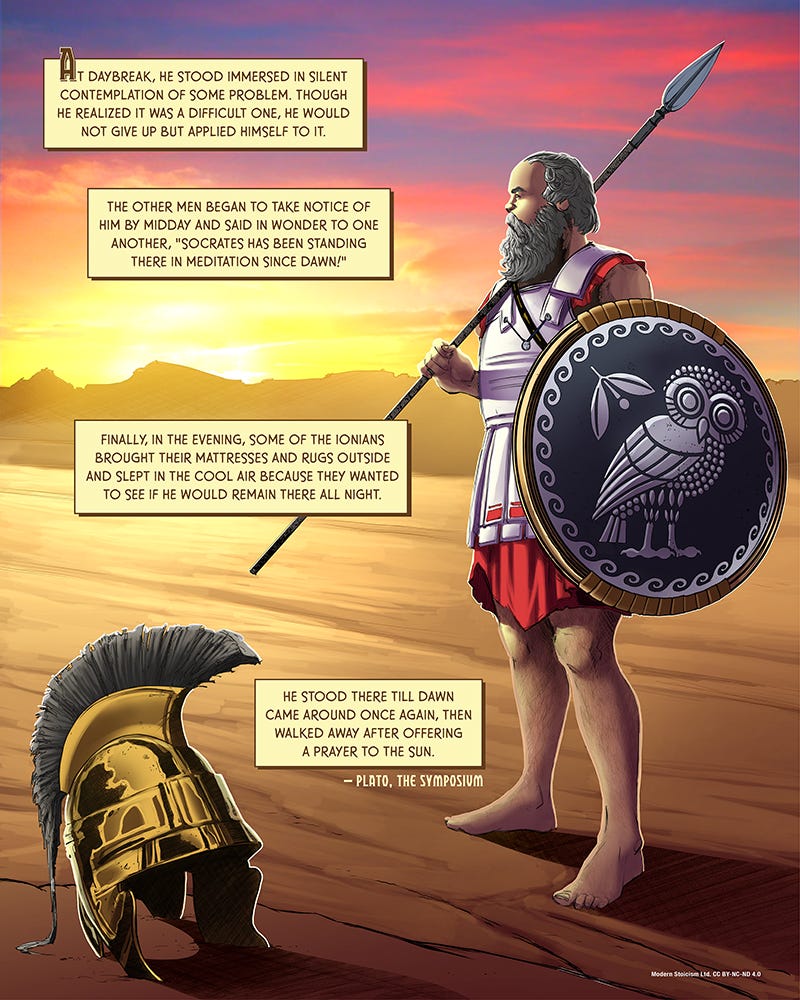The artwork is a rectangular image, approximately six inches high and four inches wide, with a portrait orientation. It features a Roman soldier or character, possibly out of a comic book, standing slightly to the right. He is depicted against a richly colored background showing a sunset over a mountainous landscape. The sunset transitions from yellows near the horizon to a gradient of reds and purples higher up in the sky. At the midline, the mountains outline provides a natural dividing line.

The soldier faces left, holding a spear with a silver tip and a brown handle in his right hand, and a round shield adorned with a white owl in his left. He wears a reddish tunic with silver armor over it and has a long beard. His helmet, positioned in the bottom left corner of the image, is golden with a distinctive black spiked mohawk.

The ground beneath him starts as dark brown packed dirt at the bottom, gradually lightening as it moves upward and left. On the left side of the image, four rectangular text boxes with a light tan or yellow background provide a narrative. The text is as follows:

1. "At daybreak, he stood immersed in silent contemplation of some problem. Though he realized it was a difficult one, he would not give up but applied himself to it."
2. "The other men began to take notice of him by midday and said in wonder to one another, 'Socrates has been standing there in meditation since dawn.'"
3. "Finally, in the evening, some of the Ionians brought their mattresses and rugs outside and slept in the cool air because they wanted to see if he would remain there all night."
4. "He stood there till dawn came around once again and then walked away after offering a prayer to the Sun. Underneath, it is signed Plato then Symposium."

Together, the visual and textual elements imbue the artwork with a sense of contemplation and endurance, drawing a parallel between the depicted Roman figure and the persevering philosopher Socrates.